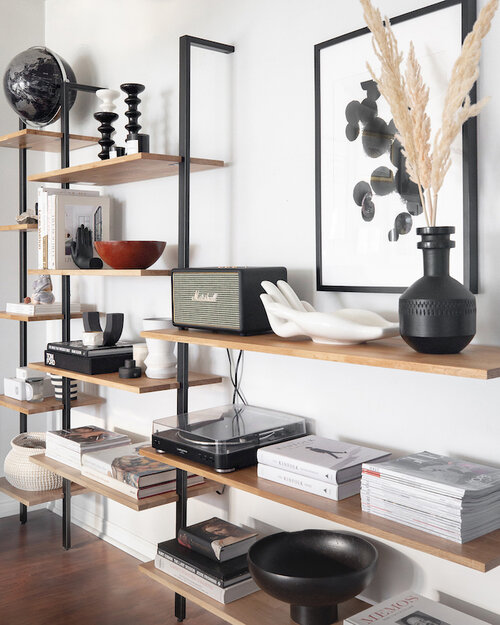The image captures a detailed, color photograph of a thoughtfully designed interior space in portrait format, showcasing a section of a modern home. The main focus is on two sets of stylized, light-colored wood shelves mounted directly onto a plain white wall with dark metal supports, exuding a vintage yet elegant theme. These shelves display a variety of carefully arranged items, including a Marshall speaker, a modern record player, a black ceramic vase, a white vase, and a red dish. Several stacks of neatly organized coffee table books in various colors and sizes contribute to the aesthetic, accompanied by an assortment of figurines, a sculpture resembling a hand, and black ceramic bookends. Additionally, there is a black globe, a bowl, and a plant with protruding leaves. A notable art piece also adorns the wall, featuring a black circular design on a white background, framed in black. The floor of the room is dark wood with a lacquer finish, providing a warm contrast to the bright, clean lines of the white wall and shelves.